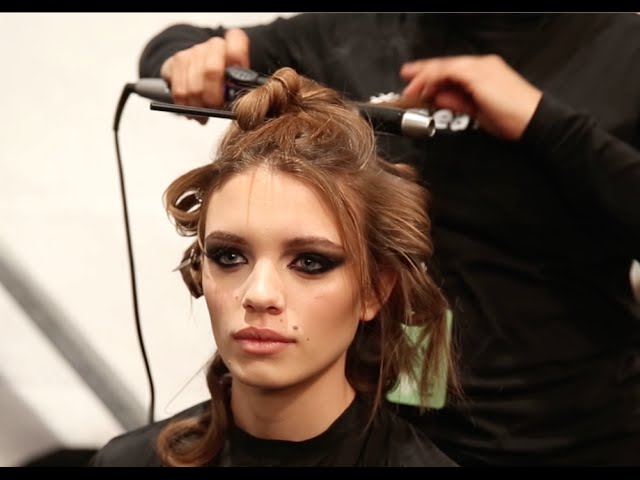In this candid backstage photograph, a model is captured in the midst of getting her hair styled. She's seated centrally in the frame, facing mostly towards the camera with her head slightly turned to the left. Her brownish-reddish hair is being meticulously curled by a hairstylist, who is dressed entirely in black. Above the model's head, the stylist's hands can be seen wielding a long, straight curling iron, with some sections of her hair also secured by additional styling tools. The model's dark, bushy eyebrows frame her light-colored eyes, which are accentuated by heavy black eyeshadow and eyeliner. Her fair skin is adorned with a prominent mole above her lip on the left side of her face, and she sports a lip-colored lipstick emphasizing her full lips. The model is dressed in a black robe, indicating a backstage setting, likely at a fashion show or similar event. Her hair and makeup are in process, exemplifying a moment of transformation before hitting the runway.